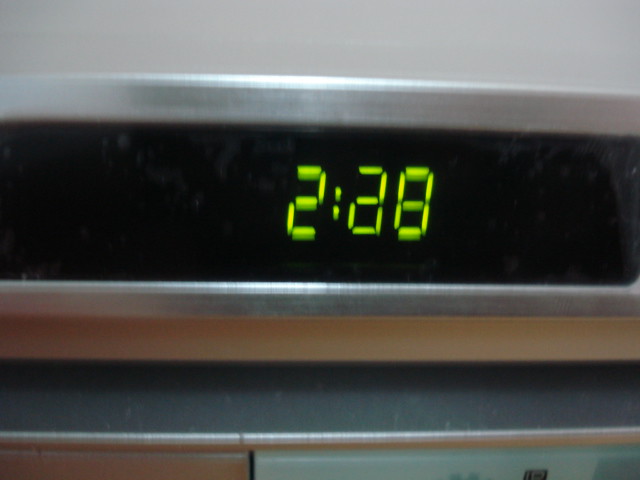The image features a close-up shot of a digital timer or clock, showcasing a rectangular black screen displaying neon green numbers "2:28". The screen is encased in a wide chrome frame with noticeable smudges, giving it a slightly dirty appearance. Above and below the screen, there are white borders, which could either be part of the appliance's facade or the surrounding wall. Below the bottom white border, a blue strip is visible, followed by another chrome border. Further down, the image captures two surfaces: one blue and the other silver, though the extreme close-up makes it difficult to discern more than their shapes and colors. On the right surface, only the top portion is visible, featuring a small black symbol. The chrome frame surrounding the black screen reflects light from an unknown source, adding to the complexity of the scene.